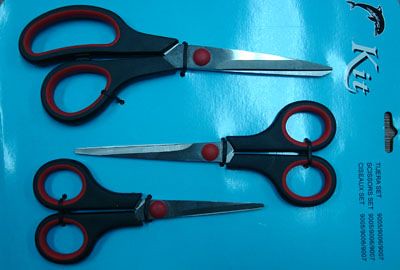This color photograph showcases a package of scissors on a turquoise blue cardboard backing. The brand name "KIT," spelled out in large white bubble letters, is prominently displayed at the top, alongside an illustration of a dolphin jumping. Beneath the brand name, there is additional writing including the words "TIJERA set," "scissors set," and "CISEAUX set," each accompanied by an inventory number, with all text oriented sideways.

The package features three pairs of scissors, each secured with small black bands and twist ties. The scissors vary in size, with one large pair and two smaller pairs. They all have rounded black handles with red interiors and are fitted with red screws that join the silver blades. The positioning of the scissors varies: the top and bottom pairs have blades pointing to the right, while the middle pair has blades pointing to the left. The package has a cutout at the top for easy hanging display. A soft glare from the lighting highlights the blue background, enhancing the overall presentation of the product.